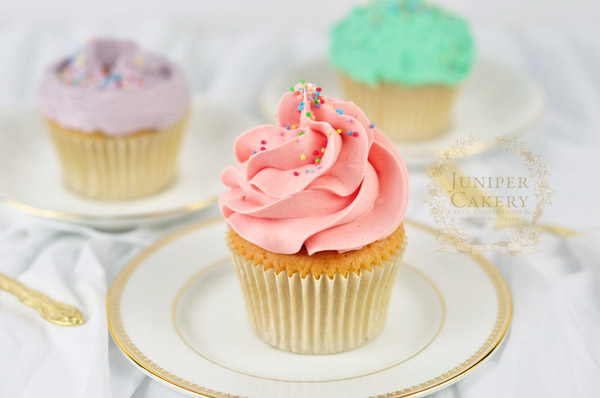This image features a sophisticated display from Juniper Cakery, showcasing an array of delectable confections and baking supplies. The logo for Juniper Cakery, positioned mid-right, is ornately designed with a golden wreath and intricate line art. The focal point of the photograph is a trio of cupcakes arranged on elegant white dishes, each accented with a gold trim. Central and most prominent is a cupcake with a golden-yellow base enveloped in a white paper wrapper. It boasts an intricate peachy-pink frosting, crowned with a delicate rose petal and sprinkled with blue, yellow, and red confetti. A finely crafted gold-plated utensil lies to the left, adding a touch of opulence. Behind this centerpiece, two additional cupcakes are artfully placed and slightly blurred: one with lush purple frosting and the other adorned with mint-green swirls, both topped with colorful sprinkles. The cupcakes sit atop a white tablecloth, which is slightly bunched to create texture, enhancing the luxurious theme of the setup.